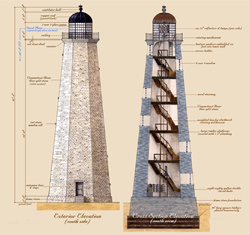This detailed blueprint features two depictions of a lighthouse against a whitish-pinkish and beige background. On the left, the external view showcases the lighthouse's solid, brick-like structure, widening at the base and tapering towards the top, resembling the shape of a salt shaker. A small door sits at the bottom of the lighthouse, with no visible windows on its column. At the top, a surrounding railing and a black exterior section for the light are visible, capped off with a roof. The right side of the blueprint provides an interior view of the same lighthouse. It reveals five distinct flights of wooden stairs that zigzag from the bottom-left to the top-left, connecting various floors and ultimately leading to the top platform. Both versions of the lighthouse are annotated with small, unreadable text and lines that detail further specifications.